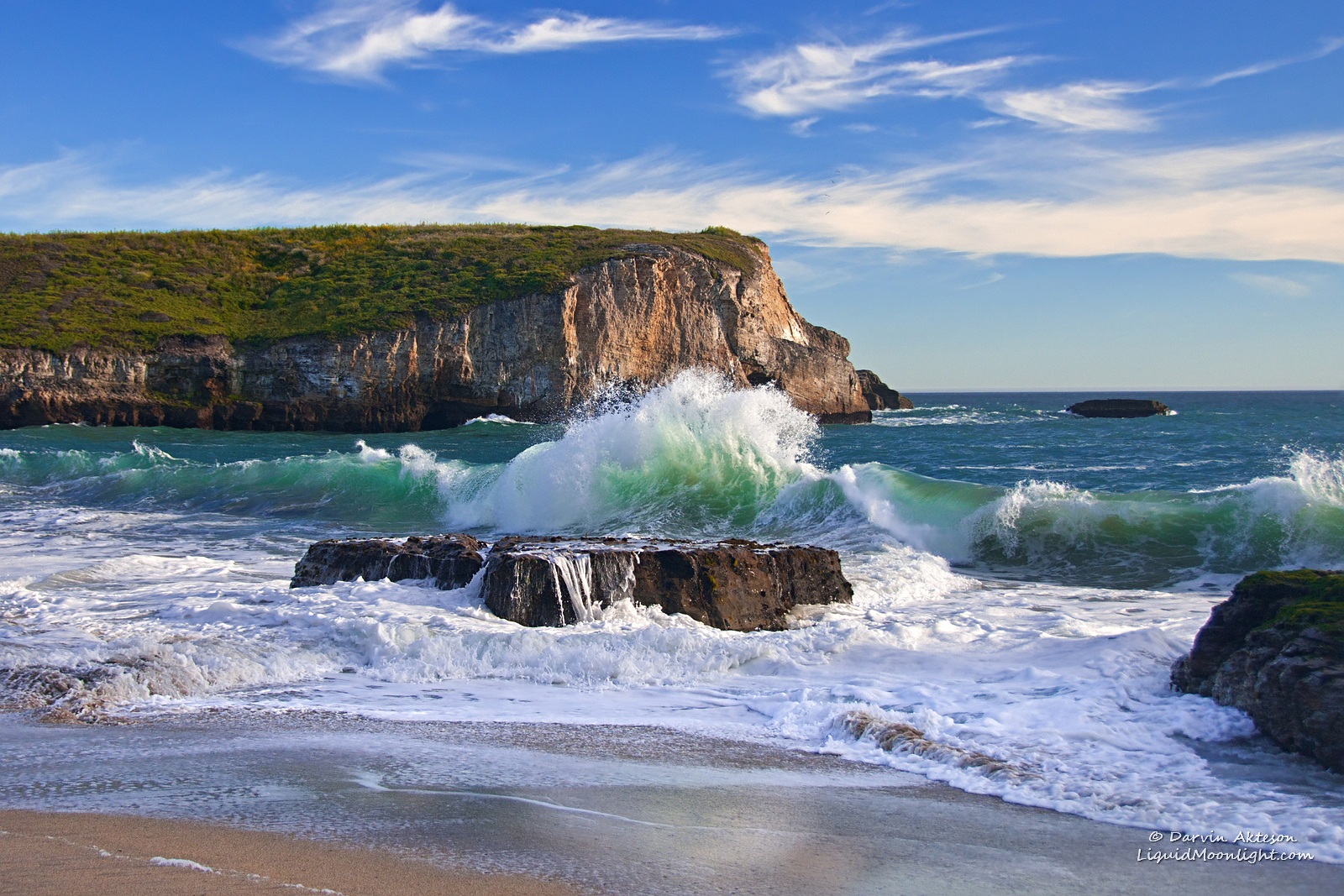The photograph captures a dynamic seascape at the beach, where high tides are rolling in energetically. Sea foam is strewn across the wet sand, evidence of the strong waves that have been hitting the shore. A particularly large wave is seen mid-crest, towering impressively as it begins to curl over. The majority of the sand is glistening with wetness due to the incoming tides.

In the foreground, large, flat-topped rocks, dark brown in color, emerge from the water. These rocks are coated with sea foam, indicating the waves continually wash over them. Beyond the tide, a lush, grass-covered mountain rises in the background, adding depth and a sense of grandeur to the scene. To the right, another object, possibly a rock, juts out from the water, adding interest to the composition.

The sky above is a blend of blue hues with a line of clouds stretching across it and a few stray clouds scattered higher up. In the bottom right-hand corner of the image, a small white font unobtrusively displays the website "liquidmoonlight.com" and the name "Darvin Atkinson."